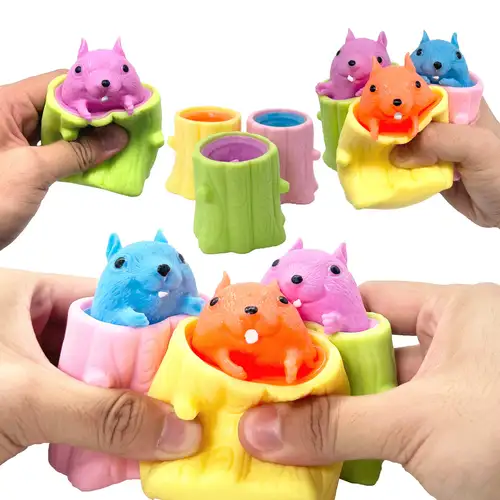In the photograph, four hands are displayed against a white background, each holding brightly colored, small toys that resemble rubber or foam tree stumps with adorable animal figures inside. The toys, vibrant in hues of green, pink, yellow, orange, light blue, and purple, are designed so that when squeezed, they reveal charming gopher-like creatures. These creatures, popping out with just their heads and little arms, boast black beady eyes, smiling faces with white buck teeth, and pointy ears. The two hands in the foreground are actively squeezing the toys, making the gophers emerge, while the other two hands in the background hold additional stumps. The scene captures the playful and tactile nature of these colorful toys as the gophers pop out from their logs with delight.